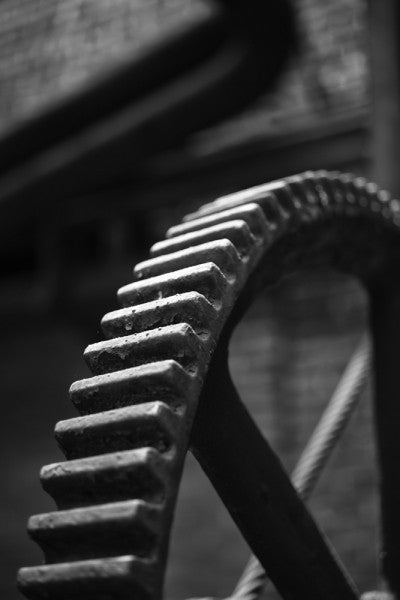The image showcases a partially visible, thin metal gear with pronounced spokes and thick, deep teeth, suggesting a piece of machinery. The gear starts its curve at the bottom left, arcs upwards toward the center, and then dips slightly as it moves toward the upper right. The gear appears tarnished and dirty, with accumulated goop between its teeth, indicating extensive use. A silver cable runs from the bottom middle to the middle right, behind the gear. The overall composition is monochromatic, with the gear exhibiting shades of gray and black. The background appears out of focus, revealing indistinct structures that resemble a wall or building.